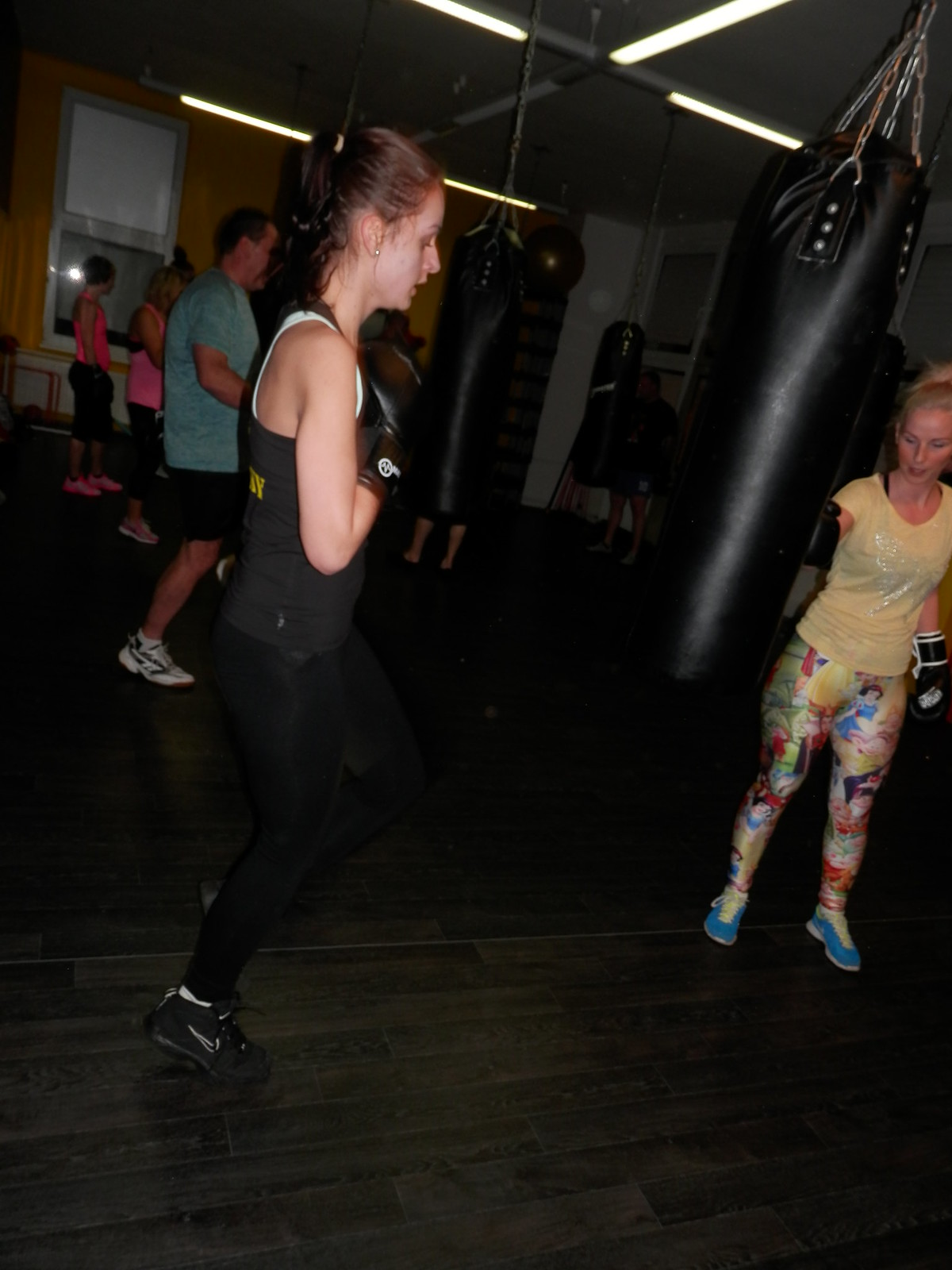In this photograph of an indoor gym, numerous individuals are participating in a kickboxing class. The wooden floor is stained and painted to appear black, and the yellow far wall is accented by a large two-pane window with a white curtain covering the top half. The white ceiling is fitted with multiple T-shaped fluorescent lighting fixtures and several chains suspending large black leather punching bags. These bags are in active use as participants engage in their training.

At the forefront, a woman dressed entirely in black—comprising a black top, tights, shoes, and gloves—is focused on a punching bag. Adjacent to her is an instructor wearing a yellow shirt, colorful patterned tights, blue shoes, and black gloves. The instructor appears to be guiding or supporting the training session. In the background, other attendees, including two women in pink, follow along with the class, each positioned in front of their own punching bags. This energetic scene captures the disciplined intensity of a kickboxing workout.